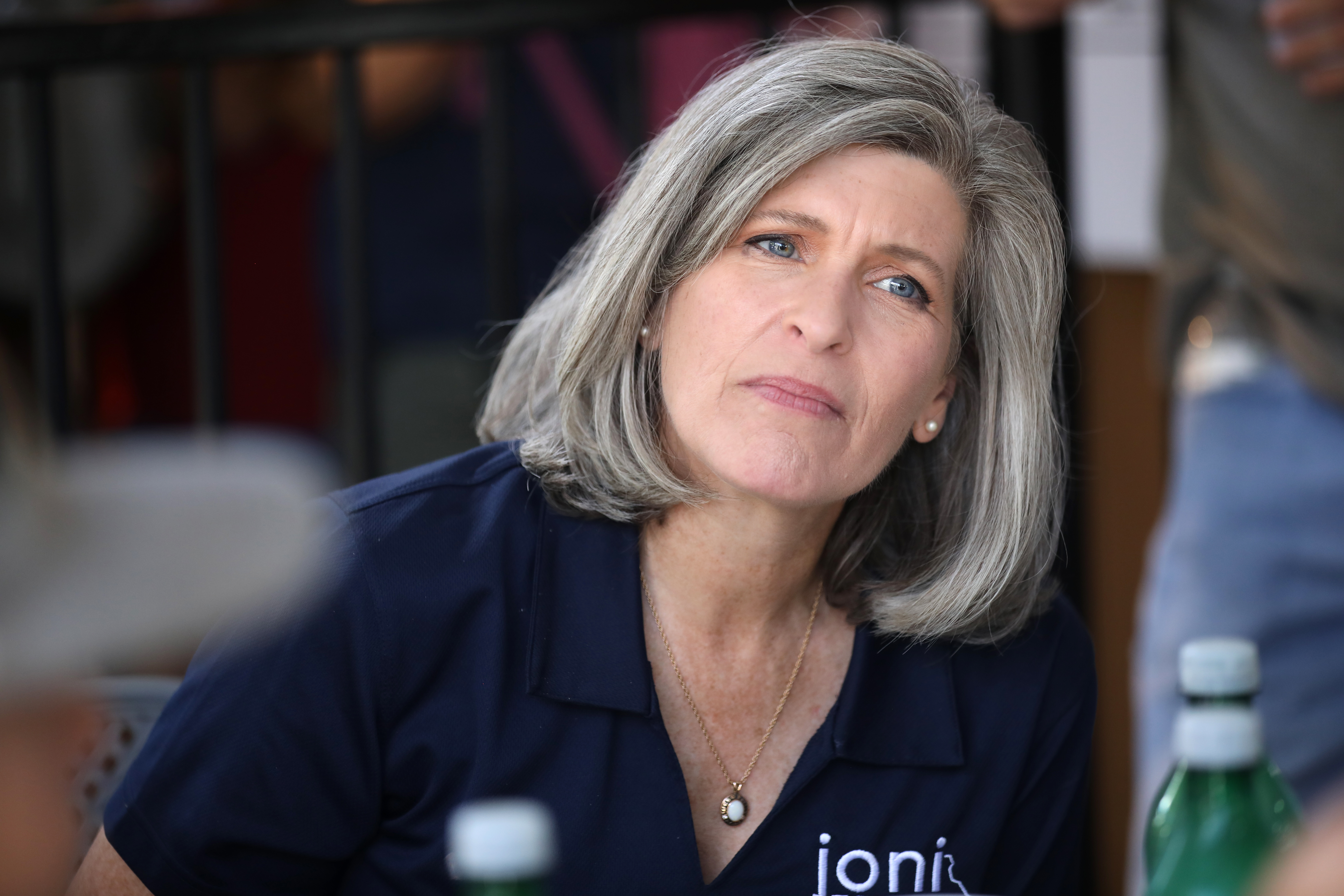In the image, a lady with shoulder-length gray hair, styled in a bob that curves underneath her chin, is seated and appears to be engaged in a conversation, looking concerned and trying to understand the other person. Her hair is tucked slightly behind her ear, and she has blue eyes highlighted by pale pink lipstick. She wears pearl earrings and a navy blue V-neck shirt with a collar, which bears the name "J-O-N-I" embroidered on the left side. Around her neck is a thin gold necklace with a white pendant, possibly a cameo. In the blurred background, there is a metal black fence. In front of her are two green bottles with lids, and to her left stands another person wearing blue jeans. A fuzzy white object is also visible towards the left side of the picture.